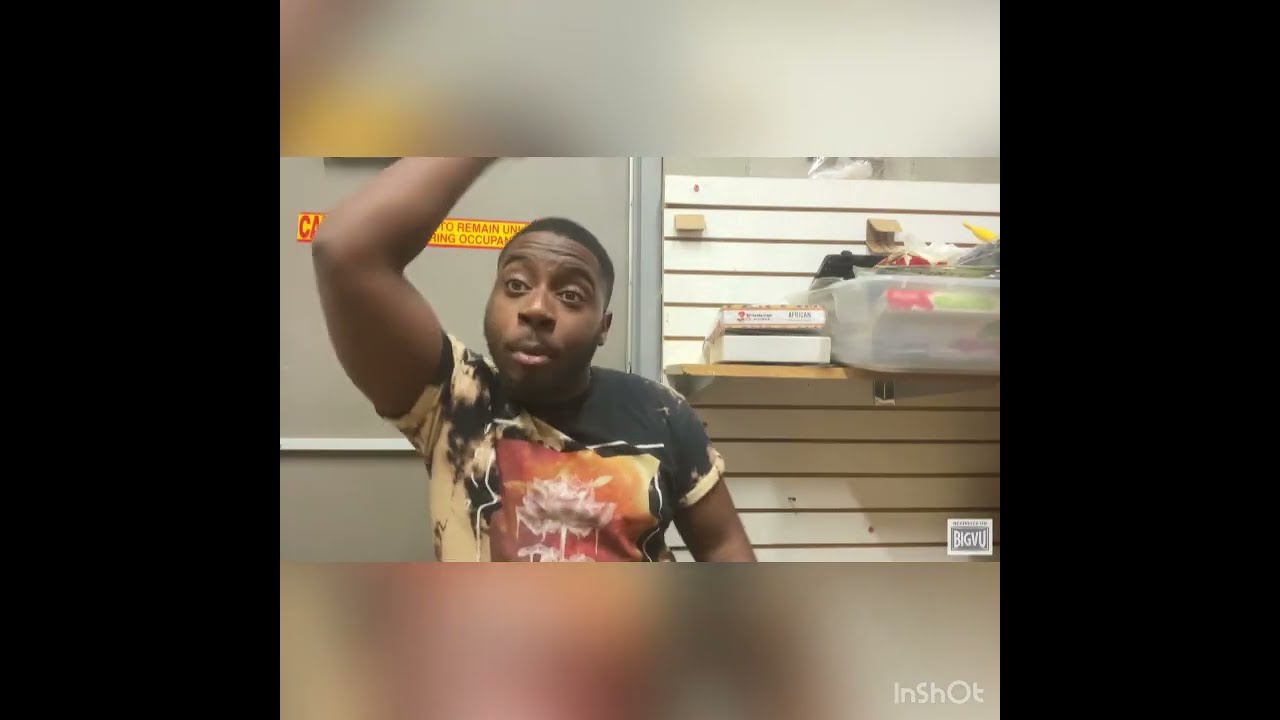The image is a screenshot taken from a video editing program, InShot, showcasing a young African American man in his mid-20s with short black hair, a trimmed beard, and a mustache. He is standing against a cream-colored pegboard-style wall with horizontal white planks and a gray security door adorned with a red and yellow caution sticker that reads "Caution, Remain" partially obscured by his raised left hand. The man is wearing a distinctive short-sleeved t-shirt that is predominantly black at the top, transitioning into hues of yellow, orange, and red, with an abstract design incorporating a pink section and an indecipherable white logo that possibly resembles an owl within a red and yellow background. Behind him, to the right of the door, there's a white wooden shelf holding a clear plastic tote filled with various items and a couple of stacked books. The image borders feature a blurred, frosted overlay of the main photograph at the top and bottom, while the sides are black. In the lower right corner, there are two logos: one gray and white reading "Big BU," and another watermark in white letters saying "InShot," reinforcing its editing program origin.